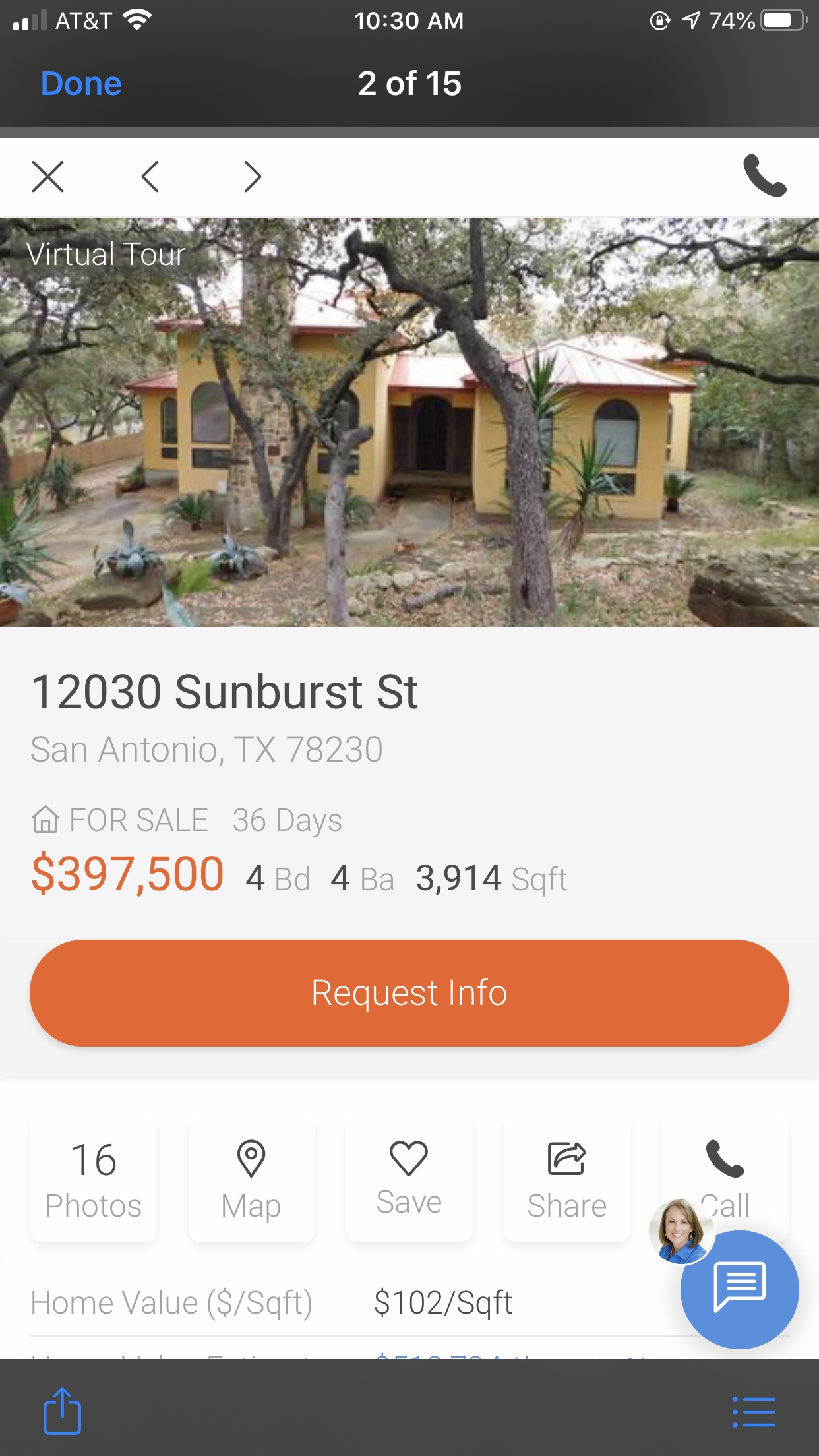This descriptive caption provides a detailed overview of the screenshot as follows:

---

The screenshot captures a detailed view of a real estate listing from a person's cell phone. Notably, the top left corner of the screen displays two bars of cellular coverage with AT&T as the carrier, connected to Wi-Fi, at 10:30 a.m., with a battery level of 74%. 

At the top, a black banner prominently features blue text reading "DONE," accompanied by a progress indicator "2 of 15". Just below, there's a vibrant photograph of a small yellow house, surrounded by a rocky landscape interspersed with sparse vegetation and framed by tall trees. A stone chimney is visible, adding to the house's quaint charm.

Directly underneath the image, the address is listed as "12030 Sunburst Street, San Antonio, Texas, 78230." The property has been on the market for 36 days, priced at $397,500. It boasts four bedrooms and four bathrooms, covering a spacious 3,914 square feet.

Below the price and description, a dark orange oblong button with white text invites users to "REQUEST INFO". Additional clickable options such as "16 photos," "MAP," "SAVE," "SHARE," and "CALL" follow.

To the right of the house listing, there is an image of a fair-skinned woman, smiling directly at the camera. Adjacent to her picture is a dark blue circle with a white text bubble icon inside.

Further details include the home value calculated at $102 per square foot, though some information at the bottom edge is partially cut off.

The bottom of the screenshot features a black horizontal banner with blue icons: one for "DOWNLOAD" on the left and a bullet list icon on the far right.

---